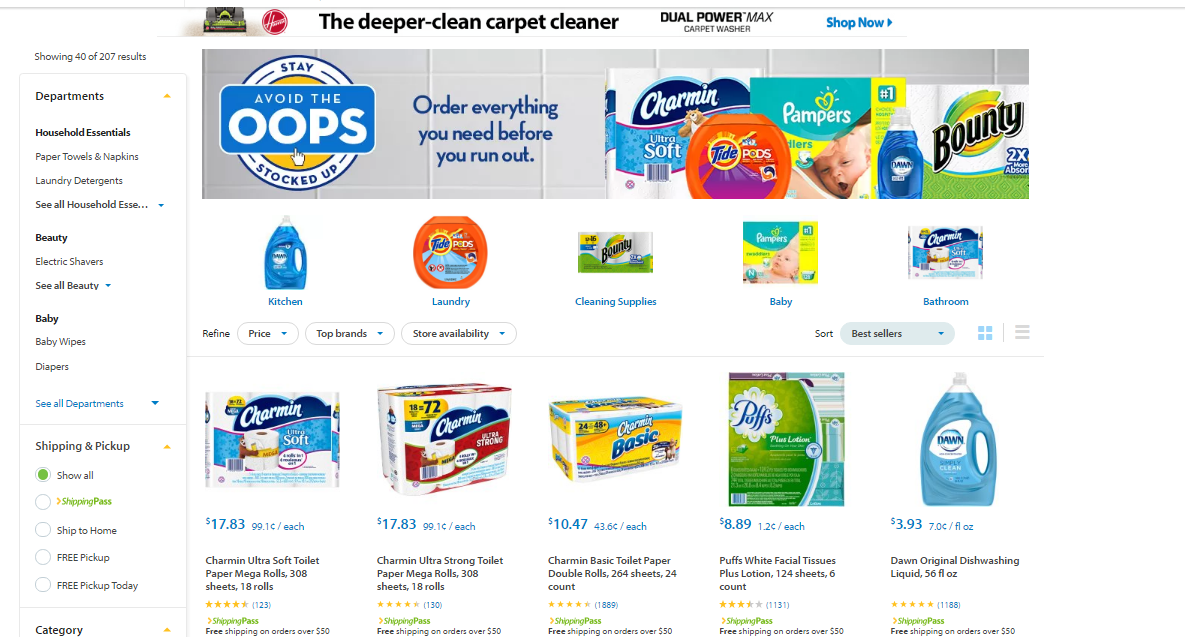The image showcases an online shopping interface highlighting the "DeeperClean and CarpetCleaner Dual PowerMax Carpet Washer." The screen displays 207 results across various categories such as Household Essentials, Paper Towels, Napkins, Laundry Detergents, Beauty products like Electric Shavers, and Baby products including Baby Wipes and Diapers. The interface provides options for shipping and pickup, with green circles indicating selectable options like shipping to home or free pickup available today.

Prominently, there's a tile on the screen with the message "Avoid the Oops, Order everything you need before you run out," emphasizing preparedness. The product listings include Charmin Ultra Soft Toilet Paper in 18-roll packs, along with other household staples like Bounty paper towels, tide laundry detergents, and Pampers baby products. Categories include Kitchen, Laundry, Cleaning Supplies, and Baby Bathroom essentials.

Overall, the image captures a comprehensive view of an online shopping experience, guiding users through product selections, shipping options, and essential household categories.